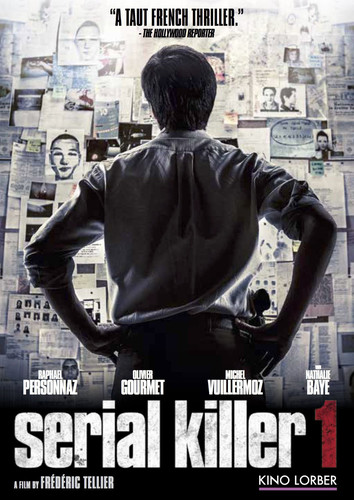The movie poster titled "Serial Killer 1" features a captivating centerpiece: a man standing in front of a bulletin board densely packed with newspaper clippings, photographs, and various articles. The man, whose back is towards the viewer, is depicted from the back of his knees up to the top of his head, wearing a white t-shirt and black pants. His hands are positioned on his hips as he scrutinizes the board. The poster's color palette includes black, white, gray, red, blue, and green tones.

At the very top of the image, black text reads, "A Taut French Thriller, The Hollywood Reporter." Below this endorsement is the man engrossed in his investigation. At the bottom of the poster, actor names are listed in white text: Rafael Personas, Oliver Gourmet, Michael Vouillemaz, and Natalie Bay. Beneath these names, the title "Serial Killer" is prominently displayed, with the numeral "1" strikingly rendered in red. Further text at the poster's bottom includes "A film by Frédéric Tellier" and "Kino Lorber" in white, situated in the bottom left and right corners, respectively. The composition of the poster effectively conveys the intense and thrilling nature of the movie.